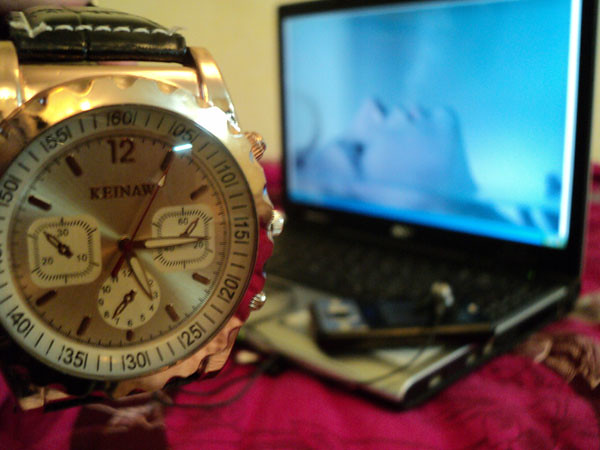The detailed color photograph displays a scene featuring two main objects placed on a red fabric surface against a light yellow background. On the left side of the image, there is an intricately designed watch. This watch has a black leather band and gold-plated latches, with a face encircled by a coppery ring and an off-white dial. The watch, marked with the brand name "KEINAW" beneath the 12 o'clock position, features brown dashes as hour marks around the circumference. The main hands, which are slightly yellow, show the time with one large hand at 15 and one smaller hand at 3, while a smaller hand points to the 5, representing the seconds. The watch face also includes three additional gauges whose purposes are unclear.

Adjacent to the watch is a laptop, identifiable by its black frame, keyboard, and silver wrist rest. The laptop's screen is blue, suggesting it is powered on. Supplementing the technological ambiance, a small gaming device sits on the laptop. The arrangement of objects provides a contrast between the warm tones of the watch and the cooler, more modern appeal of the laptop, all unified by the striking red fabric they rest upon.